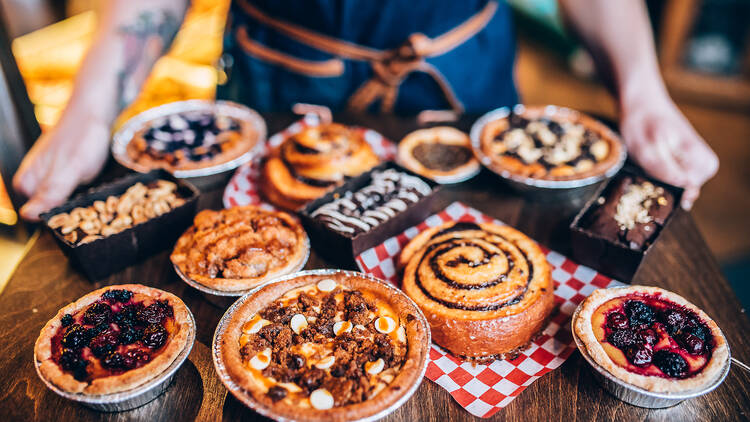In this image, a person with a tattoo on their right forearm is holding a dark wooden tray laden with various desserts. The individual appears to be wearing a blue apron with an orange or leather tie, though it might be a blue shirt. Their apron is tied at the front and they are situated in what seems to be an indoor setting. The tray features an assortment of pastries: a small pecan pie, two cinnamon rolls under a red and white checkered napkin, several small individual berry pies that could be raspberry or blackberry, a chocolate loaf cake, and a few tarts, some adorned with fruit like blueberries. Additionally, there are some cashews in a black container and other blurred desserts. The photo captures the food in sharp focus primarily at the bottom of the image, while the items and fabric details become blurry towards the top.